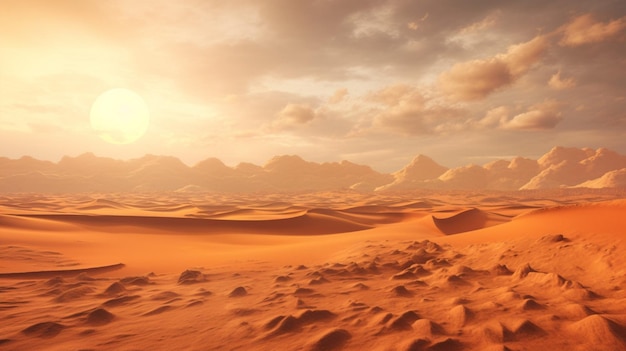This image, rendered with the style of a painting, depicts an expansive desert landscape. It features a horizontally aligned, rectangular composition, capturing the desert's intricate textures and hues. In the foreground, a medium-bright brown sand spreads across the bottom half, with wind-sculpted tiny hills and small mounds that resemble footprints. These form an intricate, almost oceanic wave pattern across the sand's surface. In the middle, the sand transitions to smoother, undulating dunes that roll from left to right, leading to larger, more prominent peaks in the background.

Stretching across the horizon, an array of low-lying mountains or dunes extends continuously from the left to the right edge of the image, painted in a light brown hue. The left-hand portion of the sky showcases a hazy sun partially obscured by light gray clouds, casting a soft, diffused light over the scene. The rest of the sky is dotted with various shades of gray and white clouds, set against a predominantly blue backdrop with hints of yellowish tones. The sun, perfectly round and bright yellow, appears to be setting, adding a subtle glow to the entire vista. The painting captures a moment of stillness in a vast, lifeless desert, devoid of water or vegetation, emphasizing the raw beauty and isolation of the arid expanse.